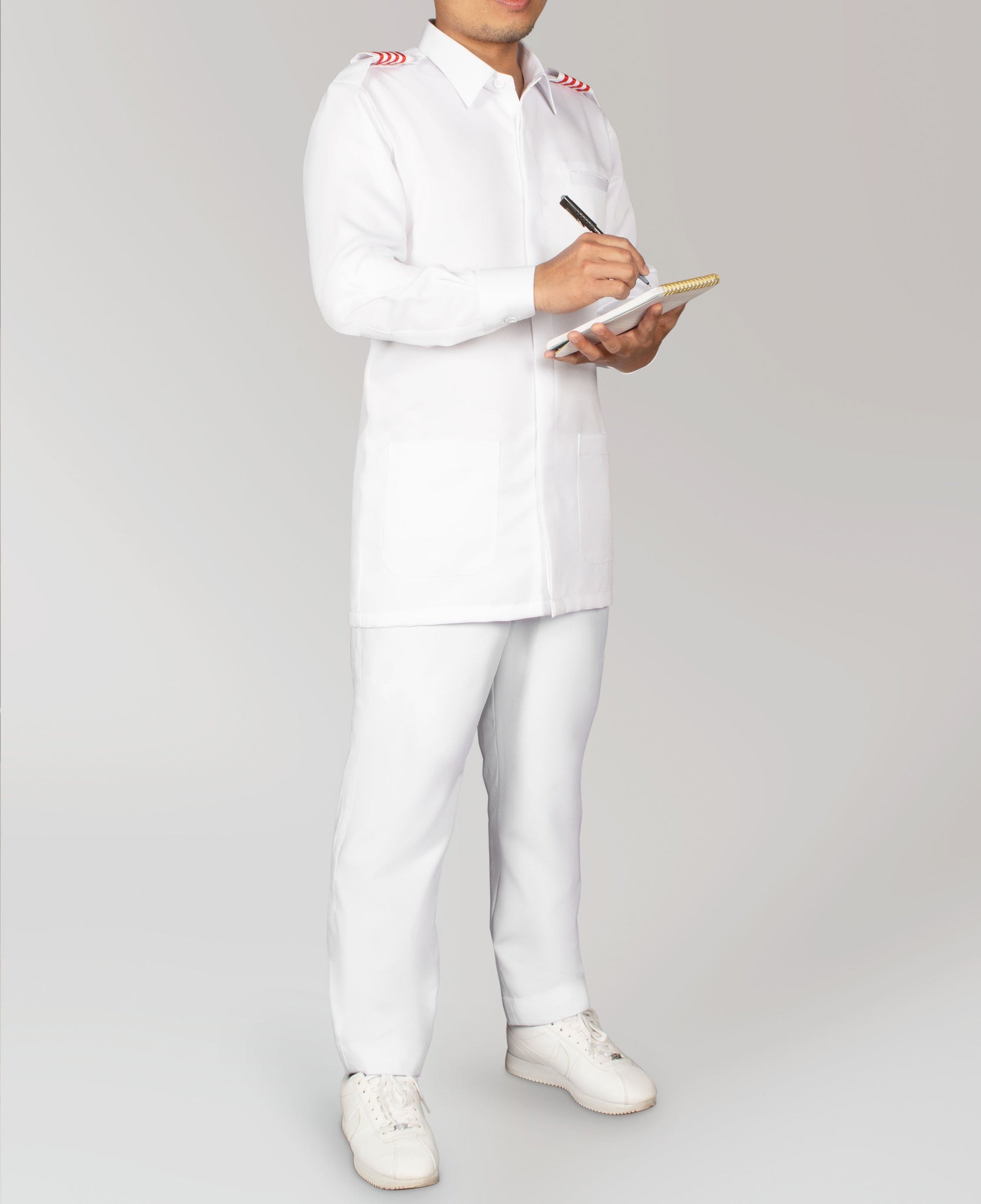The image depicts a person dressed in an all-white uniform, likely with a military or medical background, given the details and decorative elements. The individual, seen from the bottom lip down with the background in light gray, is standing vertically. The uniform includes white sneakers, white slacks, and a long white jacket featuring patch pockets and a collared, button-up design. Notably, their shoulders display three red stripes. They are holding a black pen and a white notepad, seemingly engaged in note-taking. The gray background complements the monochromatic theme of the attire. Only half of the person's head is visible within the frame of the picture.